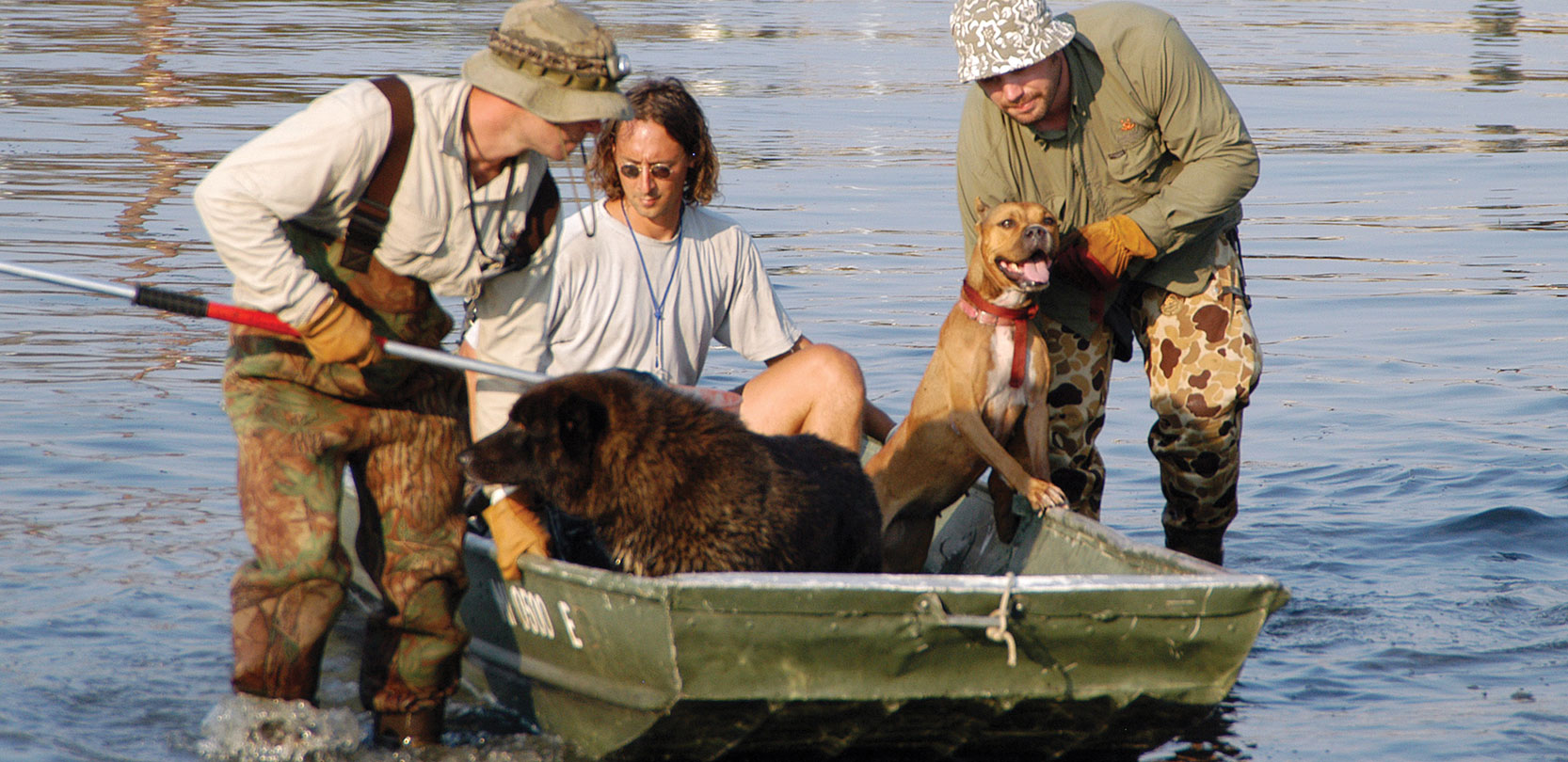This photograph captures a serene moment on the water. At the center of the image is a boat, with one man seated inside, accompanied by two dogs. The man, dressed in a white t-shirt and sporting circular sunglasses, has longer hair than the others present. The dogs beside him add a layer of charm to the scene—a fluffy canine and a possible Boxer breed, exuding a sense of companionship.

Adjacent to the boat, two men stand in the water, wearing camouflage-patterned waders and bucket hats that shield their faces from the sun. Their attire suggests they are engaged in some form of fishing or outdoor activity. One of these men is leaning towards the Boxer, petting it gently, while the other seems to be placing an item into the boat.

The backdrop of the image is a calm expanse of water, enhancing the peaceful ambiance of this idyllic outdoor scene.